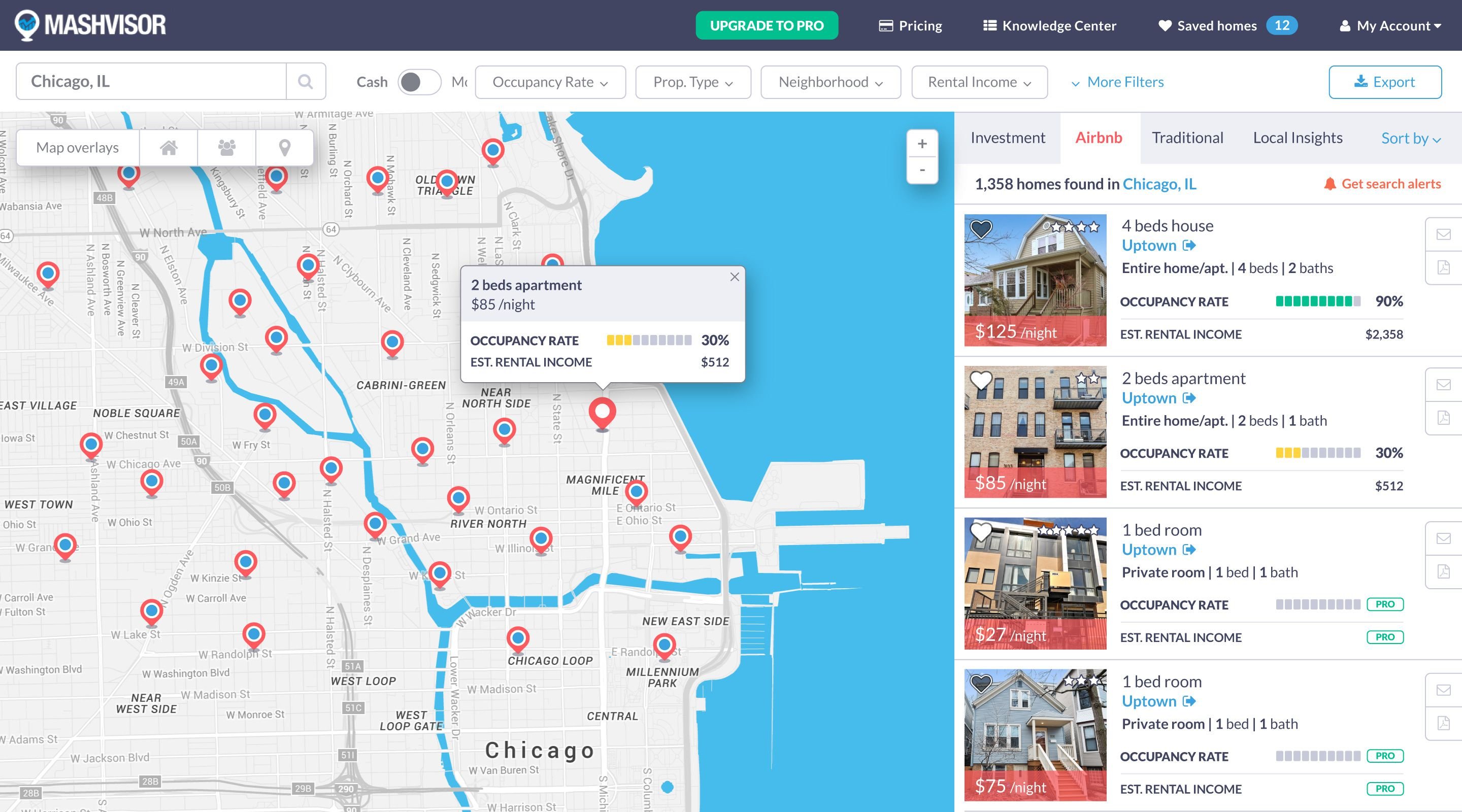This is a detailed screenshot of the MASH VISOR platform. At the top of the page, the title "MASH VISOR" is displayed prominently in all capital letters with white lettering. Navigation options including "Upgrade to Pro," "Pricing," "Knowledge Center," "Saved Homes 12," "My Account," "Chicago, Illinois," "Cash," "Occupancy Rate," "Property Type," "Neighborhood," "Rental Income," "More Filters," and "Export" are aligned adjacent to the title.

On the left side of the screen, a map of the Chicago area is displayed with a highlighted section showing specific rental information: "Two Beds Apartment, $85 per night, Occupancy Rate 30%, Estimated Rental Income $512."

On the right side, there are photographs of various homes with detailed descriptions. The first image shows a two-story house labeled "Four Beds Home, Uptown Entire Home/Apartment." It offers four beds and two baths for $125 a night, with a high occupancy rate of 90% and an estimated rental income of $2,358.

The second image features a brick apartment building with the description: "Two Beds Apartment, Uptown Entire Home/Apartment." This listing includes two beds and one bath, available for $85 a night, with an occupancy rate of 30% and an estimated rental income of $512.

The third image shows a modern-looking apartment building with a listing for a private room: "$27 a night, One Bedroom, Uptown, Private Room, One Bed, One Bath." Both the occupancy rate and estimated rental income are marked as "Pro."

Finally, the fourth image depicts a gray A-frame style house with the listing: "$75 a night, One Bedroom, Uptown, Private Room, One Bed, One Bath." Similar to the previous listing, the occupancy rate and estimated rental income are designated as "Pro."